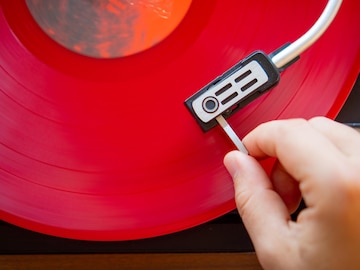An overhead close-up of a person playing a vibrant red vinyl record. In the bottom right corner, a small, well-manicured hand is delicately holding the tonearm, guiding the gold and black needle cartridge onto the spinning record. The tonearm, which is also a goldish color, arcs gracefully to the left, partially illuminated and casting soft shadows. The red vinyl reflects hints of magenta due to the lighting, which also highlights the pastel blue and orange label at the record's center. The black turntable underneath is only partially visible, adding contrast to the vivid hues above. The edge of the record player's case, made of rich wood grain, peeks into the frame, completing this richly detailed scene.